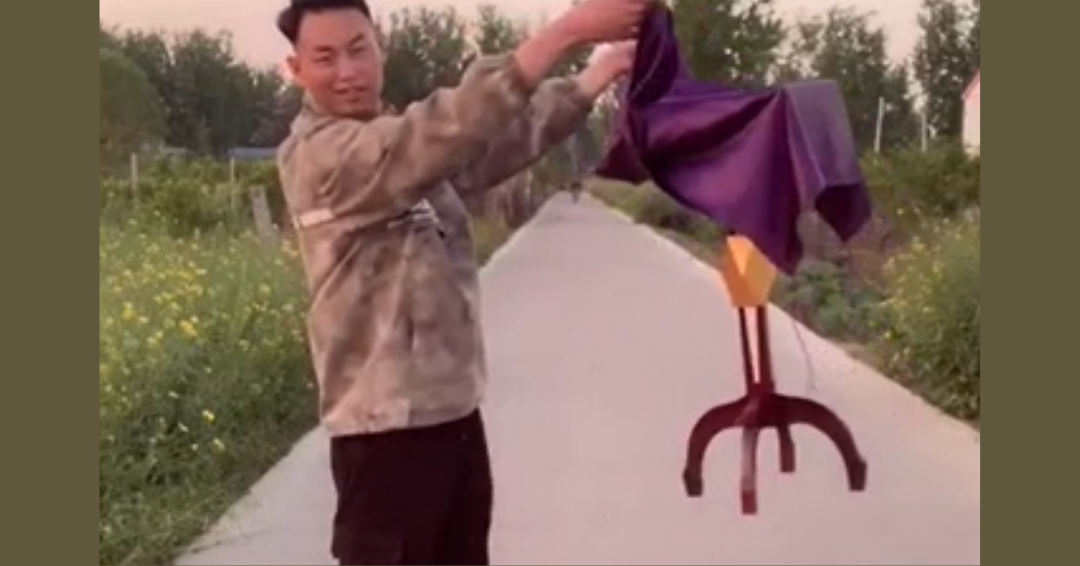In this outdoor, low-quality color photo, a man of Asian descent with short black hair is standing on a paved path bordered by green grass and yellow flowers. He gazes directly at the camera with a smirk, wearing a long, camouflaged-pattern sweater in shades of brown and white, paired with black pants. The man extends his arms forward, gripping a purple satin cloth that drapes over a table, which appears to be floating in midair—suggesting a magic trick. The table, with brown wooden legs and a golden emblem on its shaft, adds to the illusion. In the background, a blurred silhouette of a person walking can be seen. Trees frame the scene, enhancing the magical and whimsical atmosphere.